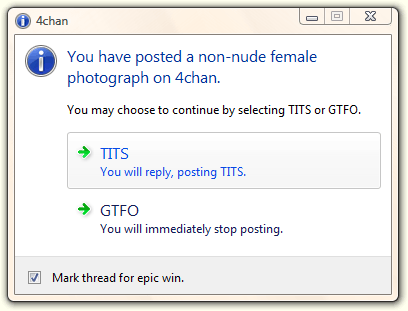The image shows a zoomed-out view of a computer browser displaying an internet meme resembling a pop-up notification on the 4chan website. At the top, there is an eye icon followed by the text "4chan." In the top right corner, there are minimize, maximize, and close (X) icons. Below this, the pop-up's title reads: "You have posted a non-nude female photograph on 4chan." It continues with a prompt in blue text, suggesting two options: "You may choose to continue by selecting TITS or GTFO." The TITS option includes a further instruction in black text: "Your reply posting TITS." The GTFO option says, "You will immediately stop posting." At the bottom of the notification, there is a checkmark inside a checkbox with the text "Mark Thread for EpicWin" inside a gray border. The background is primarily white, with light gray shading at the top and bottom.